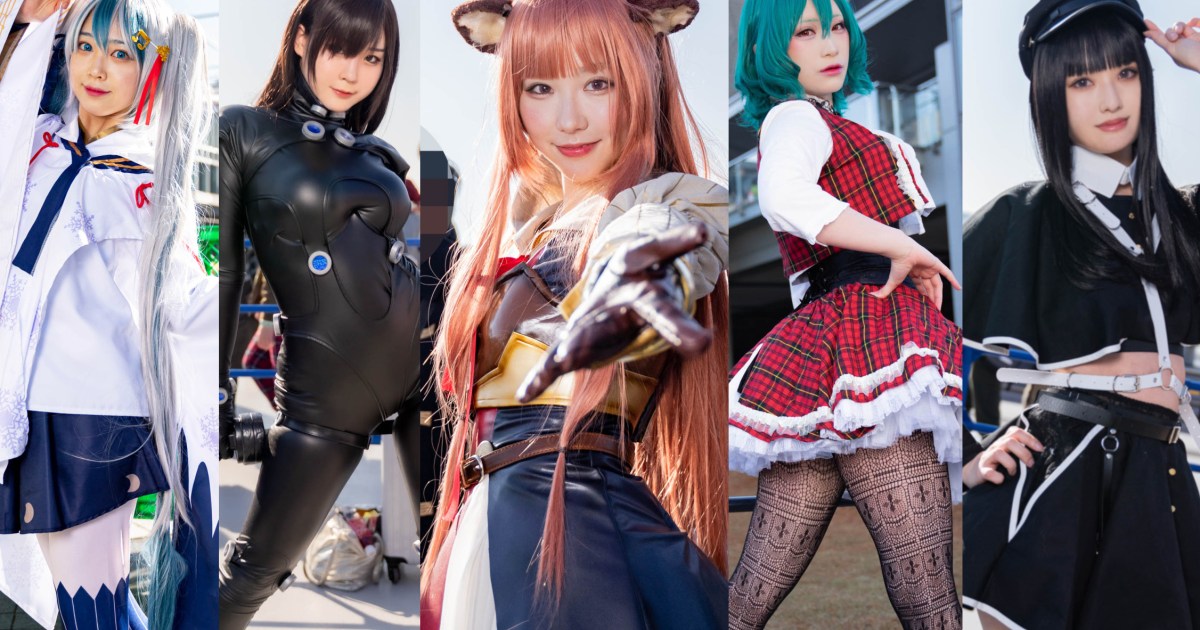The image features five different depictions of a cosplayer, neatly arranged side by side. Each segment portrays the same woman in distinct outfits, reflecting various characters and themes. 

Starting from the left, the first depiction shows her with long, white hair accented with blue streaks, wearing a schoolgirl outfit composed of a white shirt, a blue tie, a blue skirt, and blue socks. Her eyes are blue, matching the cool tones of her attire.

To the right, the second image features her in a sleek, black bodysuit adorned with blue buttons. Here she sports shoulder-length brown hair, exuding a superhero vibe as she looks directly at the camera.

The third portrait presents her with animal ears, possibly resembling a raccoon or deer, and orange-brown hair. She wears gloves and an ensemble combining a blue skirt with hints of gold and white, extending her hand forward.

In the fourth section, she appears with green hair and red eyes, dressed in an intriguing blend of white sleeves paired with a red and black plaid-patterned top and skirt, completing the look with patterned leggings.

The final depiction shows her in a sophisticated black ensemble including a hat, matching hair, and a black top with white accents that somewhat reveals her midriff. Her stance is confident, with one hand on her hip and the other seemingly about to tip her hat.

Each character portrayal highlights her versatility and attention to detail in her cosplays.